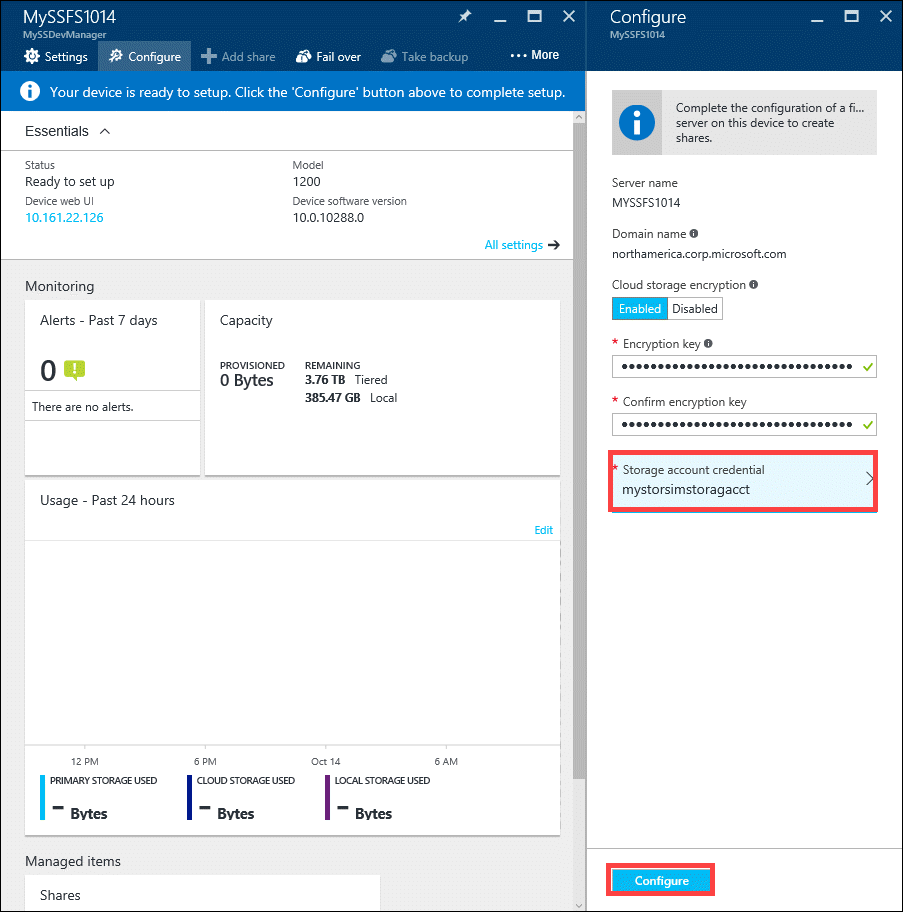**Detailed Caption:**

This screenshot is from a website titled "My SSFS 1014," specifically from a section labeled "My SSF DEV Manager." The page primarily features a white background with a striking blue header adorned with white text. The blue header prominently displays various settings options, each accompanied by a relevant icon. The options listed include "Settings," "Configure," "Add," "Share," "Fall over," and "Fake backups," with a "More" option indicated by an ellipsis.

The left side of the screen is divided into sections. Under the "essentials" section, the status is shown as "Ready to set up," along with a label "Device Work UI" followed by an IP-like address "10.161.22.125." Additionally, it provides details about the device, such as the model number "1200" and the software version number.

The "Monitoring" section reveals there have been zero alerts in the past seven days. The "Capacity" section indicates zero bytes used with 3.7 terabytes remaining in a tiered structure. Below, the "Usage Past 24 Hours" section displays zero bytes used across primary storage, cloud storage, and local storage.

On the right side of the screen, there is a prompt to "Complete the configuration of the server of this device to create shares," providing the server name "mysfs1014" and the domain name "northamerica.corp.microsoft.com." Additionally, there are inputs for "Cloud Storage Encryption" and "Confirm Encryption Key," both obscured for security. A "Configure" button is positioned at the bottom of the screen.